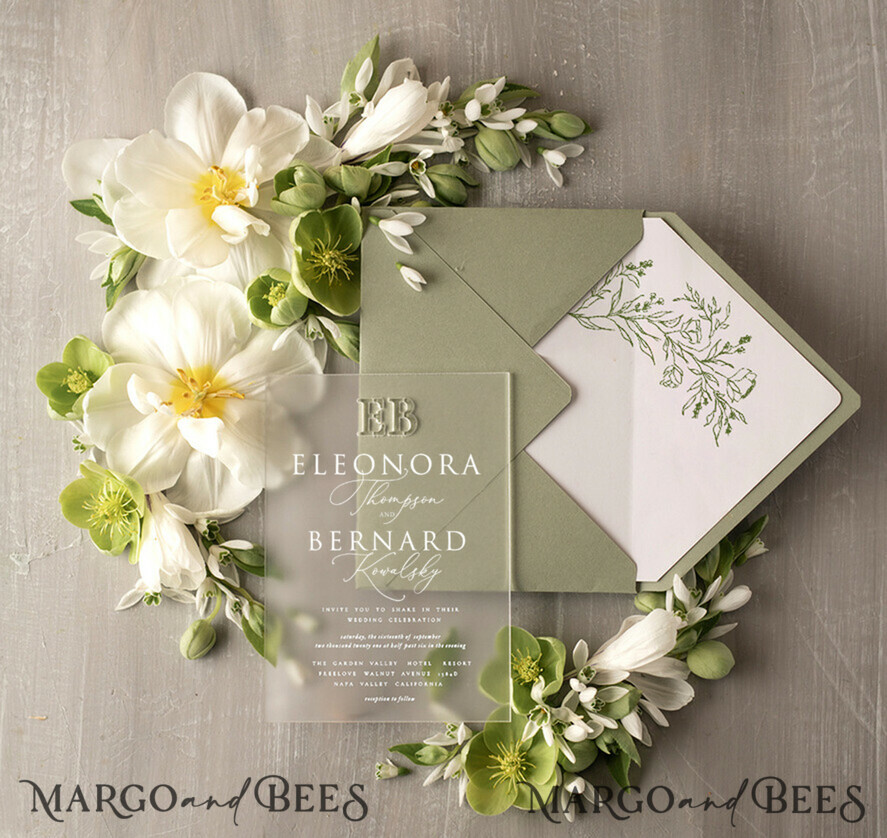This beautifully crafted advertisement for Margot and Bees showcases an elegant wedding invitation set against a rustic, grey clapboard-patterned table. At the forefront, an open green envelope reveals a white liner adorned with intricate green floral designs. Displayed atop the envelope is a clear invitation inscribed with gold lettering reading "E.B." and elegantly scripted details for the union of Eleonora Thompson and Bernard Kelsey. Surrounding the invitation is a charming garland of white flowers with yellow centers, interspersed with small green blooms and lush greenery. At the bottom of the image, in stylish cursive-like print, the brand name "Margot and Bees" appears twice, affirming the company's craftsmanship and attention to detail.